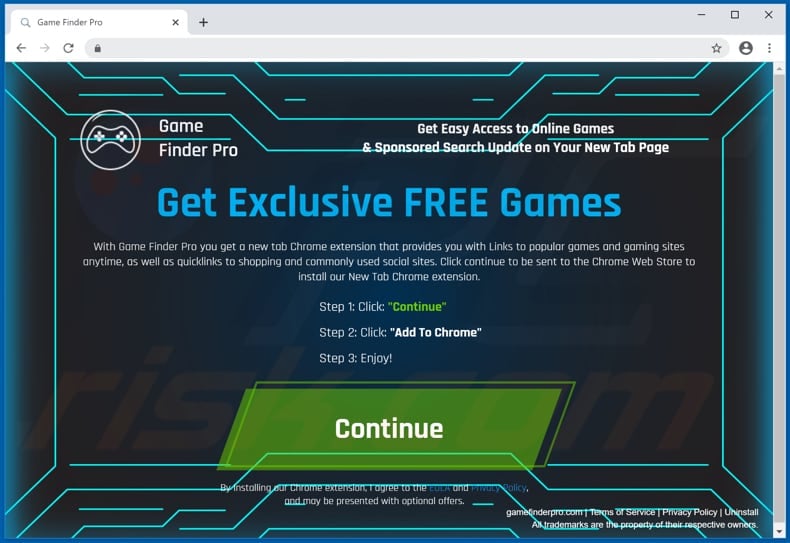### Detailed Caption:

This image is a screenshot of a single-tab browser window displaying the "Game Finder Pro" website. The browser interface includes standard navigation elements: minimize, maximize, and close buttons in the upper right corner, all encompassed within a navy blue border. An address bar is centrally located at the top, featuring a favorite star icon at its far end and a user avatar to the extreme right. To the far left of the address bar are standard browsing icons: a back arrow, a forward arrow, and a refresh button.

The main content area showcases the "Game Finder Pro" website, prominently positioned slightly to the left. The site’s logo, depicting a game controller with a white outline, is visible. Below the logo, the company name is displayed in blue text alongside a tagline: "Get exclusive free games."

The webpage guides users through three steps, each detailed as follows:
1. "Click 'Continue'" - The word "Continue" appears in quotation marks and is highlighted in green.
2. "Click 'Add to Chrome'" - This instruction is also in quotation marks with "Add to Chrome" in white text.
3. "Enjoy"

A slanted green "Continue" button is prominently displayed at the bottom of the page.

Stylistically, the website has a futuristic Tron-like design, characterized by glowing blue lines and accents against a dark blue, almost black background. Above the "Get exclusive free games" tagline, a small white section reads: "Get easy access to online games and sponsored each update on YouTube tab page."